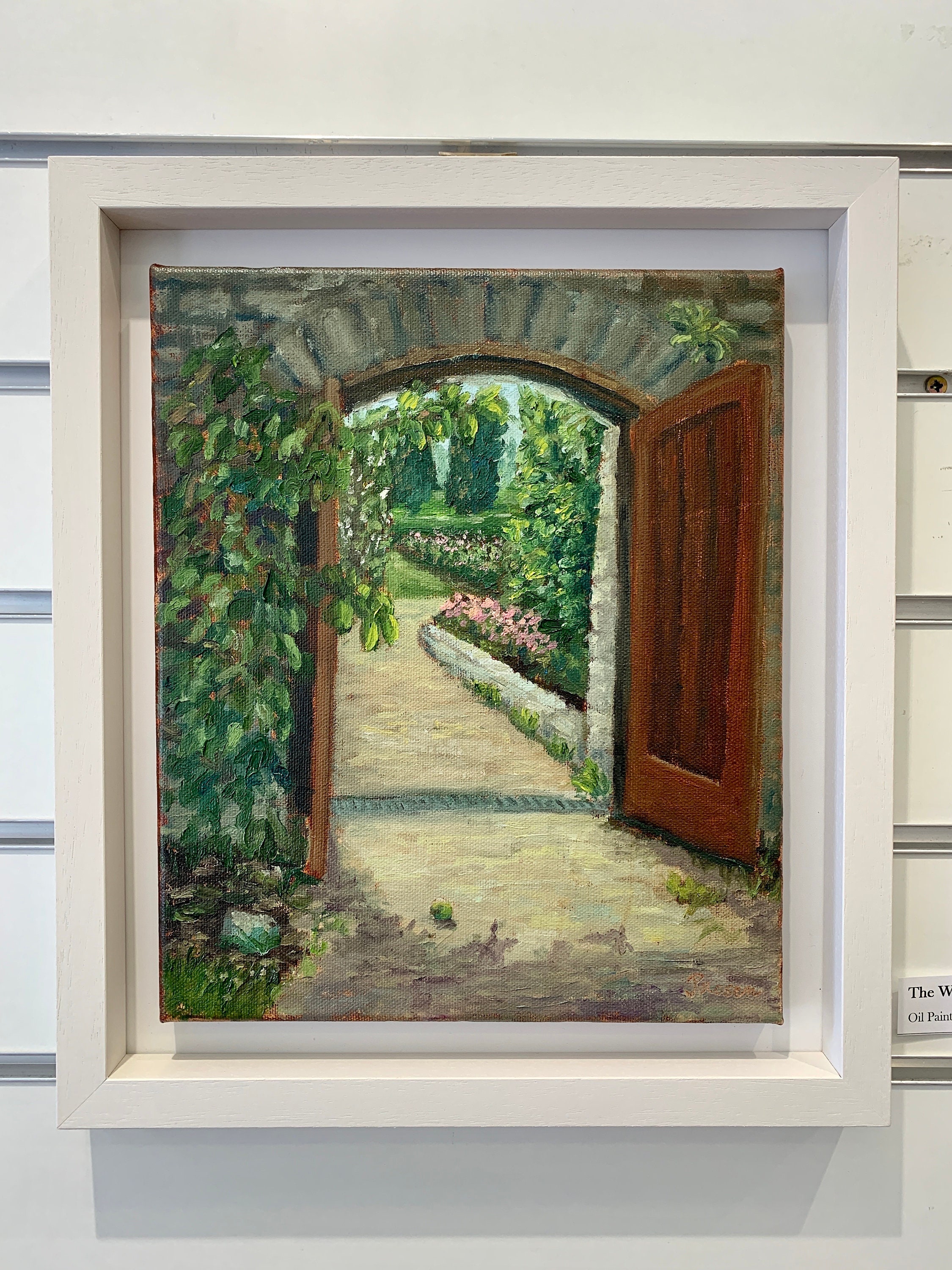This full-color image depicts an oil painting elegantly framed in a white rectangular vertical frame, hung on a wall made of white horizontal wooden planks with slight gaps in between. The framed painting itself has a thin white border. Inside the painting, a stone archway with an open wooden door invites the viewer to step into a beautifully manicured garden. The arch and the door are framed by gray brick, with green ivy climbing up the left side. Beyond the doorway, a dirt path meanders through the lush garden, lined with vibrant green bushes, trees, and pink flowers, suggesting a serene, idyllic environment. In the bottom right of the image, a small horizontal piece of paper with black text identifies the painting, indicating it’s an oil painting titled "The W". No artist's name is visible.